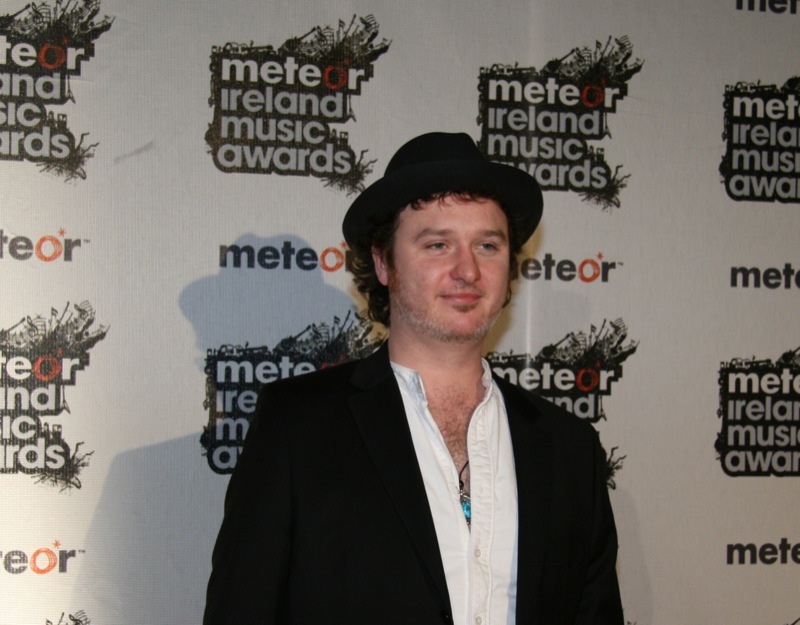In this detailed and descriptive caption, we integrate shared and repeated details from all descriptions:

The color photograph captures a man, appearing to be around 35 years old, standing alone and posing at the Meteor Ireland Music Awards. He sports a stylish black top hat and a black suit jacket over an open-collared white shirt, through which a hint of a turquoise necklace peeks out. His curly hair slightly pokes out from under the hat, and he has some facial hair, including a bit of gray in his mustache and beard, giving him a youthful yet distinguished look. He is positioned towards the center bottom of the landscape-oriented image, casting a shadow to his left. The man stands in front of a white backdrop adorned with repeating logos. The logos read "Meteor Ireland Music Awards" with alternating rows displaying the word "Meteor" alone. The "O" in "Meteor" is orange and slightly distorted, accompanied by a star symbol, evoking the imagery of a meteor in space. He faces slightly to the right with a half-smile, embodying the quintessential image of a musician prepared to perform.